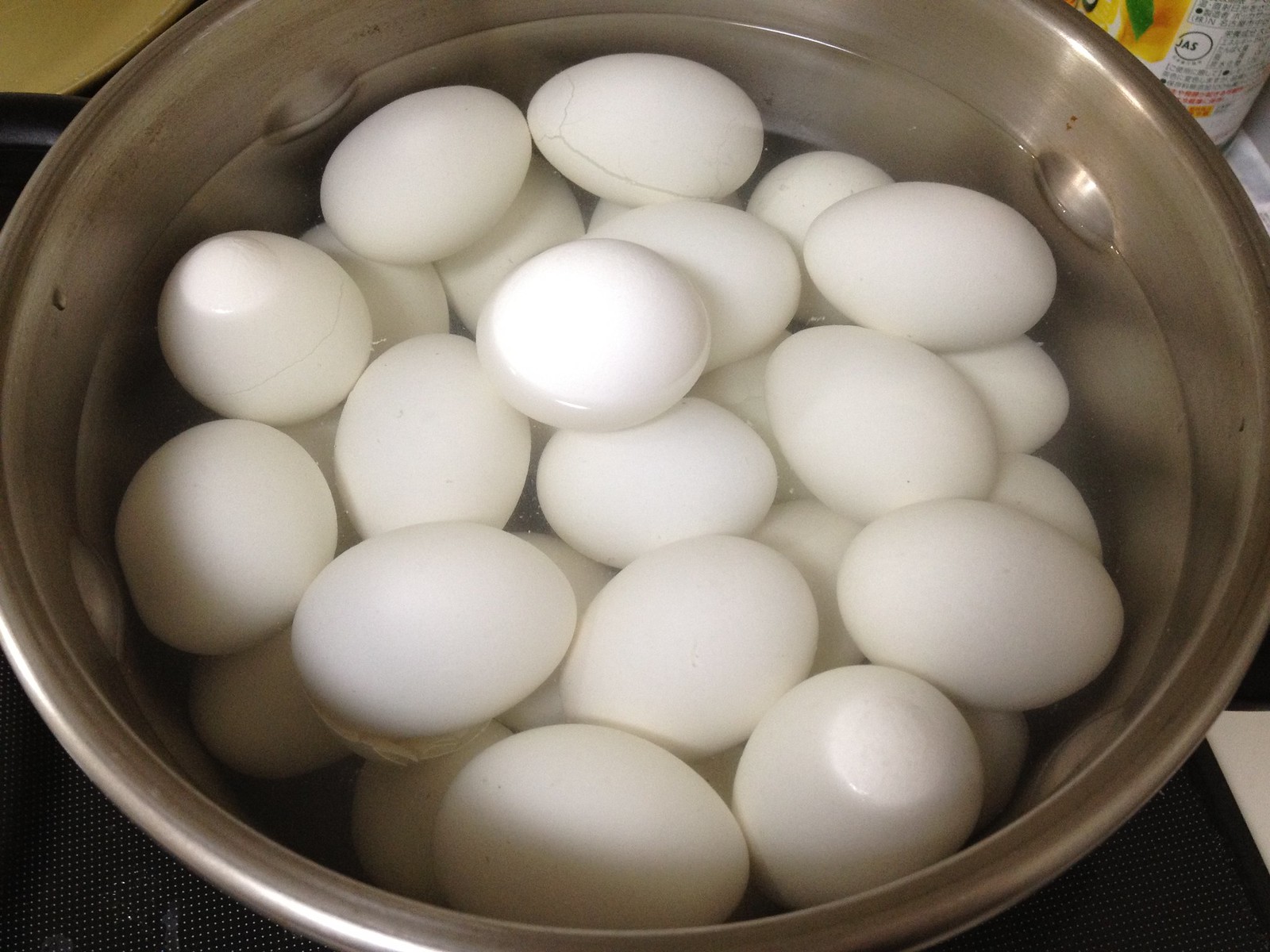The photograph features a large, stainless steel mixing bowl filled with a substantial quantity of white eggs, estimated to be around two to three dozen, mostly submerged in water. Some of the eggs exhibit visible cracks, suggesting they have been hard-boiled. The bowl, deep and round, is positioned on a black surface that appears to be covered with a textured, netting-like fabric. In the upper right corner of the image, a beverage can or bottle with Chinese characters and a graphic of an orange or yellow fruit, accompanied by a green leaf, is partially visible, adding a subtle yet distinct background detail.